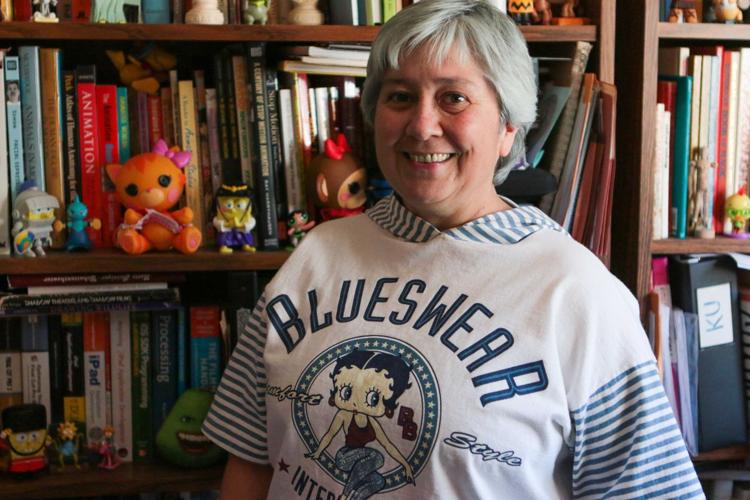A cheerful older woman, perhaps in her 60s, stands contentedly in front of an elaborate bookshelf filled to the brim with a multitude of books and various small, colorful figurines. Her white hair, short and slightly swooped over her forehead, frames her bright, smiling face with dark eyes and eyebrows. She's dressed in a cozy-looking oversized white sweatshirt with blue stripes on the collar and elbow-length sleeves. The sweater proudly displays an illustration of Betty Boop donning a red sleeveless shirt and blue jeans, encircled by white dots on a blue background, labeled "Blues Wear" with the words "comfort" and "style." Her pleasant demeanor adds warmth to the scene, enhanced by a bookshelf decorated with whimsical plastic figures of animals and other characters, including a pig, a cat, and what appears to be a goldfish, contributing to a lighthearted and charming atmosphere.